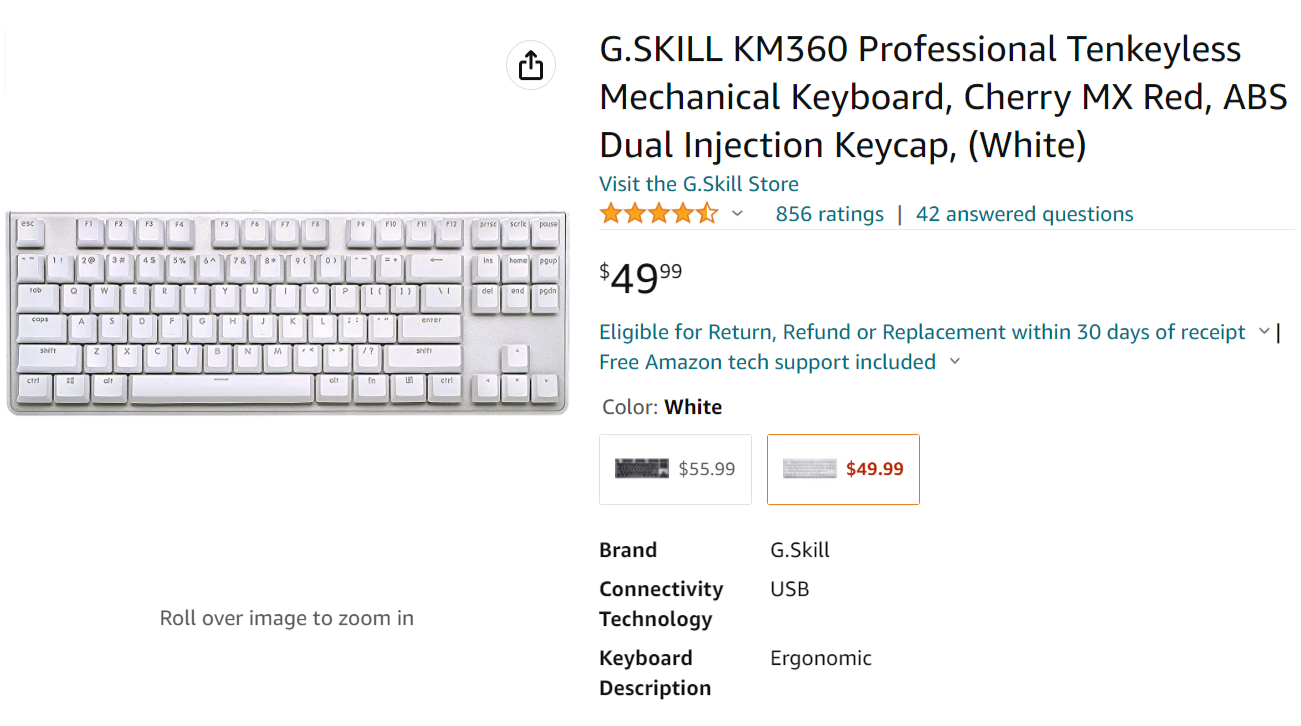This image showcases a detailed advertisement for a computer keyboard, possibly resembling an Amazon listing. The ad is divided into two sections. On the left-hand side, there's a high-resolution picture of a white keyboard, identified as the G.Skill KM360 Professional Tenkeyless Mechanical Keyboard. The keyboard is noted for its spacious layout, featuring prominently displayed and well-spaced function keys, which are larger than standard keys. The ergonomic design and overall aesthetic of the white keyboard are clearly visible.

On the right-hand side of the image, the product description is meticulously detailed. It states the full name of the keyboard: "G.Skill KM360 Professional Tenkeyless Mechanical Keyboard Cherry MX Red ABS Dual Injection Keycap," with "white" specified in parentheses to denote the color. This section mimics the format of a typical product description found on an e-commerce platform, including hyperlinks to the G.Skill store and user ratings. Below the description, the price is listed, accompanied by an option to choose a black version of the keyboard, which is available at a higher cost. The ad is informative and user-friendly, providing all essential details at a glance.